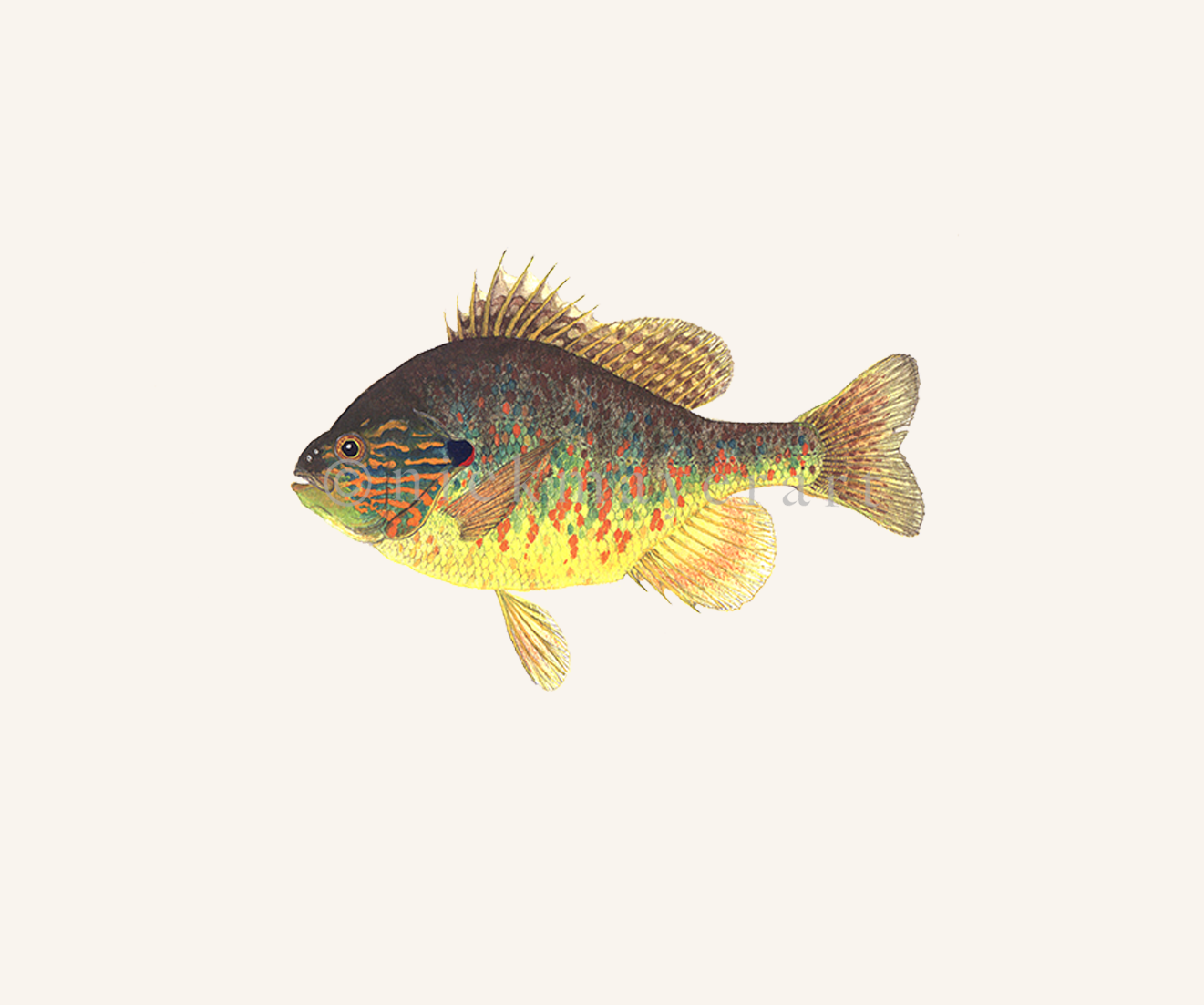This illustration depicts a stocky, oval-shaped fish against a plain, light beige background, with ample white space surrounding it. The fish is oriented to the left, with its mouth open. Its thick body is widest at the middle and tapers towards a smaller, fanned-out tail. The fish features a vibrant yellow belly that transitions into hues of blue-green and dark gray, almost black, at the top. Its upper body exhibits a mix of reds, greens, oranges, and some blues, with some red lines branching from its face near the gill.

The fish has two prominent fins at the top of its body; the first, located at the forward section, is spiky and composed of elongated spines, while the second, smoother fin, extends toward the tail. The tail fin is unsplit and features brown spots. At the bottom, the fish has two yellow and orange fins. A small, brownish-yellow fin is also present on the back of its body, adding to its colorful appearance. The fish's dark eye and rounded appearance indicate it's a lively species, resembling panfish such as perch or bass, although this is merely an illustration and not a real fish.